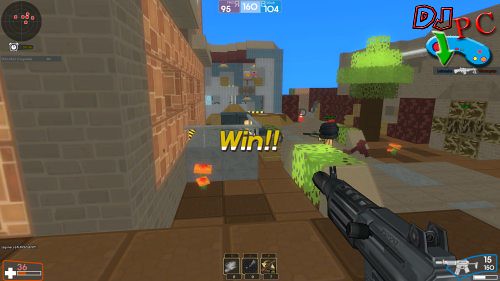In this high-intensity scene from a first-person shooter game, the player's perspective is keenly illustrated. The environment is rich with detail, showcasing a maze-like corridor composed of buildings with brick and stone surfaces. The colors vary from earthy browns to cool grays, with the bricks under scattered sunlight and shadows, adding depth to the setting. The player appears to be cautiously navigating the passage, peeking around corners in anticipation of hidden threats.

Dominating the foreground is an immense gun, emphasizing the shooter's readiness. On the left side of the screen, two glowing squares draw attention, possibly indicating power-ups or interactive elements. Boldly displayed just above the gun is the exclamation "WIN!!," suggesting a recent victory. The upper right corner of the image features the text "DJ PC," potentially the player's username or a gaming tag. The scene is void of other characters, focusing instead on ambient details and possible pick-ups signaled by small, illuminated squares scattered through the frame.